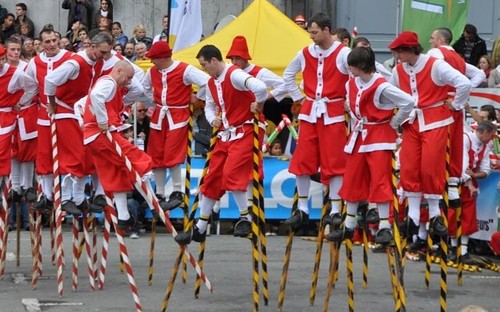This image captures a vibrant festival or parade scene set outdoors. A group of men, dressed uniformly in red knee-length shorts and red tops with white trim and red buttons over white long-sleeved shirts, stand impressively on stilts. Their footwear consists of knee-high white socks paired with black clogs. The stilts vary in design, with some being striped red and white, while others are black and yellow. Among the stilt-walkers, three men wear distinct hats, two of which match, and one that is longer. 

In the lively background, a yellow canopy and assorted flags are visible above a grey wall and a half fence. Crowds gathered behind the barricade, which sections off the grey road occupied by the stilt-walkers, suggest a festive atmosphere. The crowd's presence, along with the playful interaction of two men clashing their stilts together, emphasizes the celebratory and communal spirit of the event.